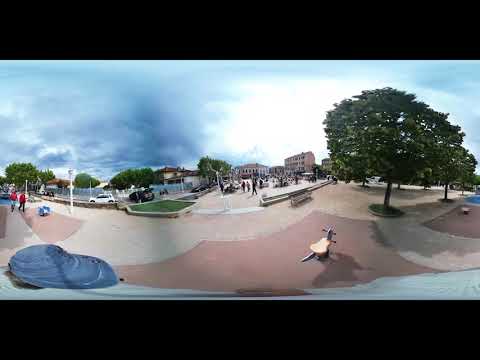The image captures a vibrant outdoor scene on a bright, slightly cloudy day in what seems to be a large park or community gathering area. Dominating the front and center is a bustling skate park, replete with rails and numerous people engaged in various activities such as skating and walking. The park's flooring has a distinctive light red, almost adobe hue. On the left side of the image, a small parking lot features a white car and a black car, and parked cars line the street. Two people, easily recognizable in their red shirts and black pants, are walking towards the center. Trees border the right-hand side and patches of grass are interspersed throughout the area. The sky above is a rich blue, with clouds that appear slightly gray on the left, hinting at possible rain. Far in the background, brownish buildings with black windows stand prominently. Various benches are scattered around, providing spots for relaxation. Despite being a 360-degree image, which blurs some finer details, the overall scene buzzes with life and community activity.